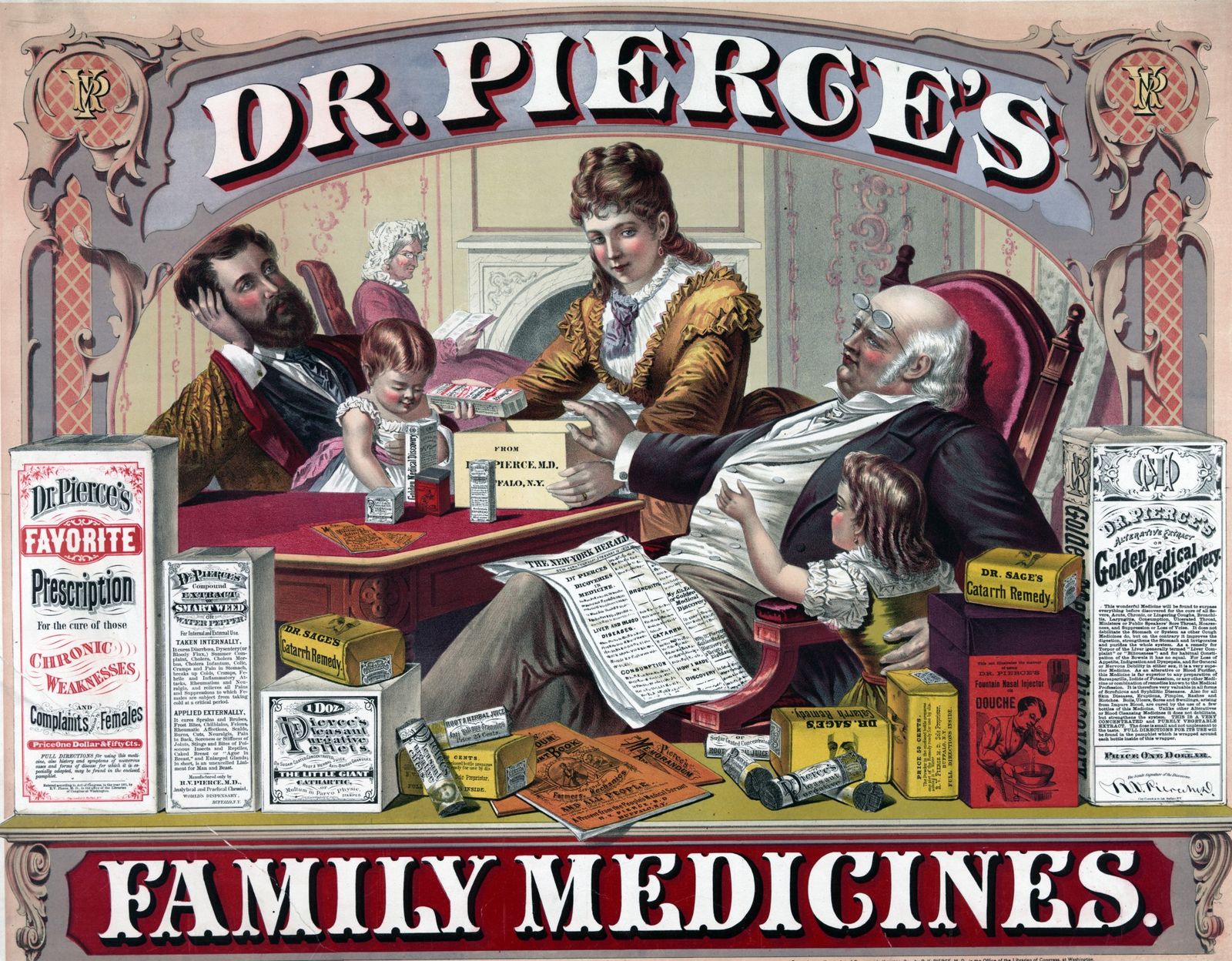The image is a colorful, vintage-style advertisement for Dr. Pierce's Family Medicines, prominently displaying the text "Dr. Pierce's Family Medicines" at the top. It appears to capture a 19th-century family scene as viewed through a window, suggesting an intimate glimpse into a family home and their everyday life. The family members are dressed in period-appropriate Victorian attire, including a woman with brown hair, a man with a beard, and a balding elderly man with white hair and glasses, all gathered around a red table. An old grandmother is seen in the background, sitting in a red chair and reading a book.

The advertisement features various products around the scene, such as newspapers and orange booklets labeled "Golden Medical Discovery" and other items mentioning "Favorite Prescription, Chronic Weaknesses, Complaints Females." It is filled with boxes, papers, leaflets, and tubes, organized to convey the array of available medicinal products. The illustration emphasizes the nostalgic, familial, and homey setting, reinforcing the idea of trusted family remedies from a bygone era.